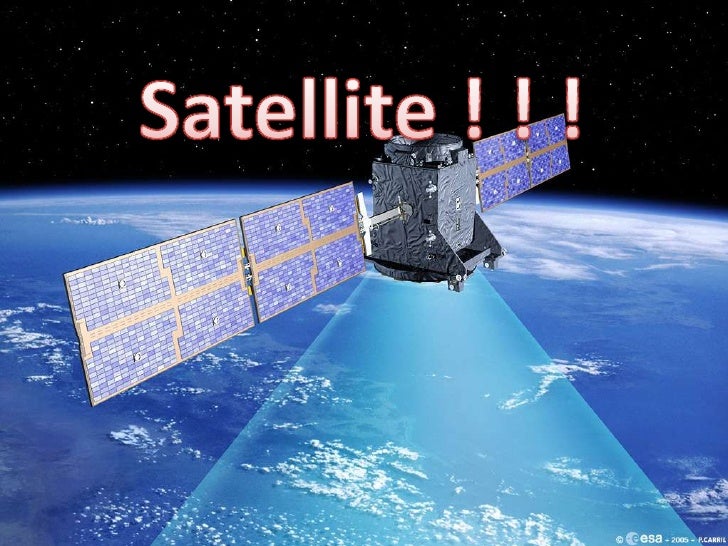The image depicts a computer-rendered satellite orbiting in outer space. The satellite, which has a square-shaped body in shades of dark and light gray, features two arms on each side adorned with panels that are an intricate mix of blue, white, gray, and purplish hues. These panels appear to be solar cells. From its underside, a bright turquoise beam emerges, directed towards the planet Earth. The Earth below shows a deep blue expanse of oceans interspersed with white clouds, capturing the visual contrast vividly. The background above the satellite is the blackness of space, dotted with twinkling white stars. At the top of the image, the word "satellite" is prominently displayed in white with a red outline and punctuated by three exclamation points.